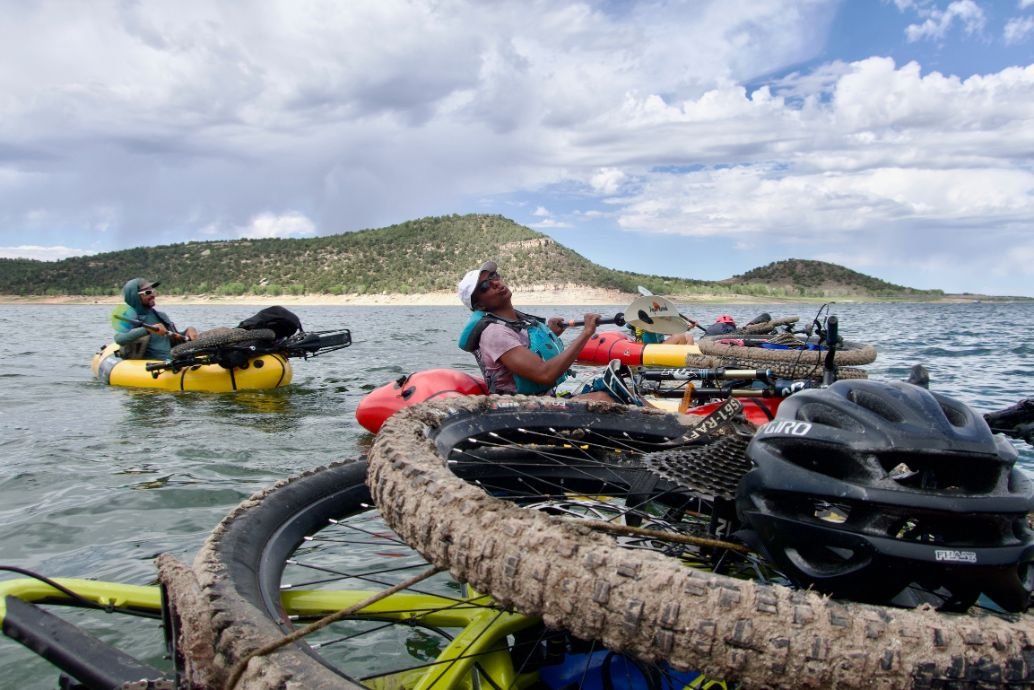This outdoor adventure picture vividly captures a thrilling moment during what seems to be a multi-sport event, likely involving triathletes. The scene is set against a backdrop of a clear blue sky dotted with white clouds, and a lush, green hill. In the background, a water body—possibly a river or sea—stretches out, reflecting the clear sky. In the foreground, several athletes are prominently visible, paddling on small, inflatable rafts. 

The athletes, adorned in caps, T-shirts, safety jackets, gloves, and helmets, are meticulously prepared for their journey. They are transporting their bicycles, which includes both dirt bikes and cycles, loaded atop the rafts, indicating either a transition between segments of the race or preparation for the next phase. The close-up of bike wheels and helmets in the bottom right corner of the image adds depth and focus to the narrative.

In total, up to five rafts are discernible, with athletes actively rowing and coordinating their movements. The captured moment is from the point of view of one of the riders, providing an immersive experience. The gentle slope of the green shrub-covered hill and the visible beach in the background enhance the adventurous and rugged ambiance of the picture.